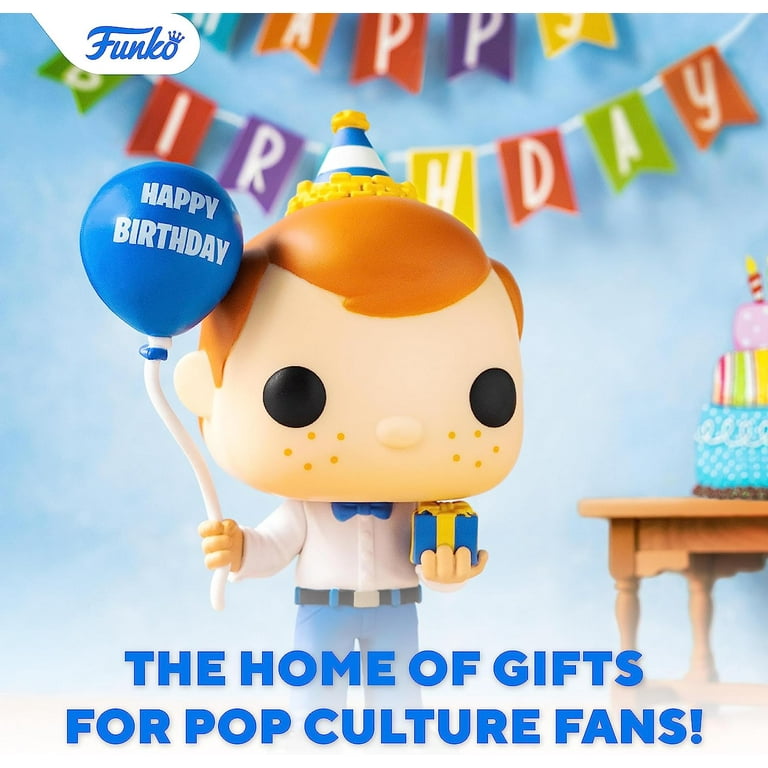The image is a square-shaped poster, likely designed for a platform like Instagram, showcasing a central Funko Pop character. The character is a young boy with a disproportionately large head compared to his body, featuring solid black eyes and a small button nose. His light cream-colored skin is accented by little yellow freckles under his eyes. He has red hair that's parted to the left and is shorter on that side, allowing his ears to stick out clearly. Atop his head, he wears a blue and white striped conical party hat with a yellow tip and a yellow ring at the base, resembling small bricks.

He is dressed in a white button-down shirt, blue bow tie, blue jeans, and a black belt. In his left hand, he holds a string attached to a blue balloon that says "Happy Birthday" in white text. In his right hand, he holds a white gift box adorned with blue and yellow accents. The poster also shows a wooden table with a three-layer cake on the right side. The cake layers are decorated with various colors and patterns: the bottom layer is blue with spirals, the middle layer has vertical lines in red, green, and yellow, and the top layer is pink with white dots, topped with a red and white candle.

At the top left corner of the poster is the blue Funko logo on a white background. A "Happy Birthday" banner arches across the top with multicolored letters: blue, orange, red, green, yellow, purple, and more. At the bottom of the poster, large blue text reads, "The home of gifts for pop culture fans."